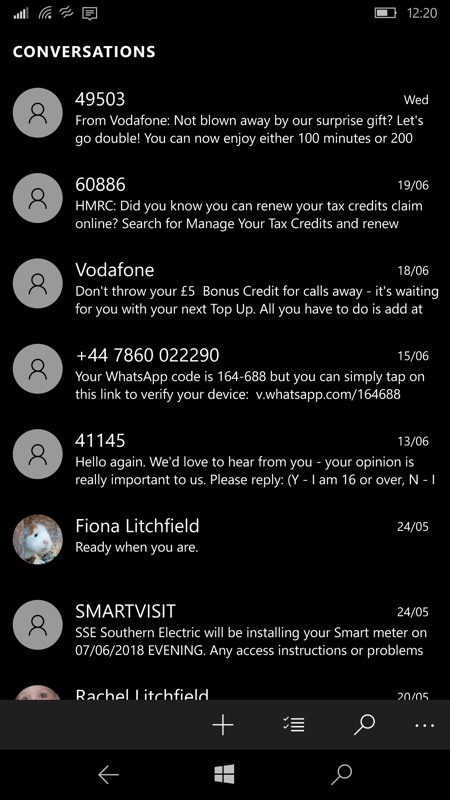Screenshot of Windows Device Displaying Conversations

This image is a screenshot captured from a Windows phone or tablet. The user interface at the bottom features navigational elements including a left-pointing arrow, the Windows logo, and a magnifying glass icon. Just above these, there are icons for a plus sign, a checklist with check marks, another magnifying glass, and three horizontal dots, likely for additional options. 

The top of the screen shows the device's status indicators: four out of five bars for cellular signal strength, a grayed-out Wi-Fi icon, a grayed-out icon resembling curvy waves, and a grayed-out text bubble icon. The battery level is approximately 75%, and the time displayed is 12:20.

The main portion of the screenshot presents a series of conversations. Most profiles use a generic placeholder image. The messages visible include:

1. From 49503 Vodafone: "Not blown away by a surprise gift? Let's go double. You can now enjoy either 100 minutes or 200..." (Wednesday)
2. From 60886 HMRC: "Did you know that you can renew your tax credits claim online? Search for 'manage your tax credits and renew.'" (June 19)
3. From 49503 Vodafone: "Don't throw away your five euro bonus credits for calls. It's waiting for you with your next top-up. All you have to do is add..." (June 18)
4. From 44786002290 WhatsApp: "Your WhatsApp code is 164-688. Tap this link to verify your device: v.whatsapp.com/164688." (June 15)
5. From 41145: "Hello again. We'd love to hear from you. Your opinion is really important to us. Please reply 'YES I am 16 or over' or in case you are under 16..." (June 13)
6. Fiona Litchfield with a mouse or hamster icon: "Ready when you are. Our visit from SSE Southern Electric will be installing your smart meter on June 7th, 2018 evening. Any access instructions or problems..." (May 24)
7. Rachel Litchfield (profile image appears to be a child): "520" (May 20)

The conversations reveal various automated messages, reminders, and notifications related to services such as Vodafone, HMRC, WhatsApp, and SSE Southern Electric.